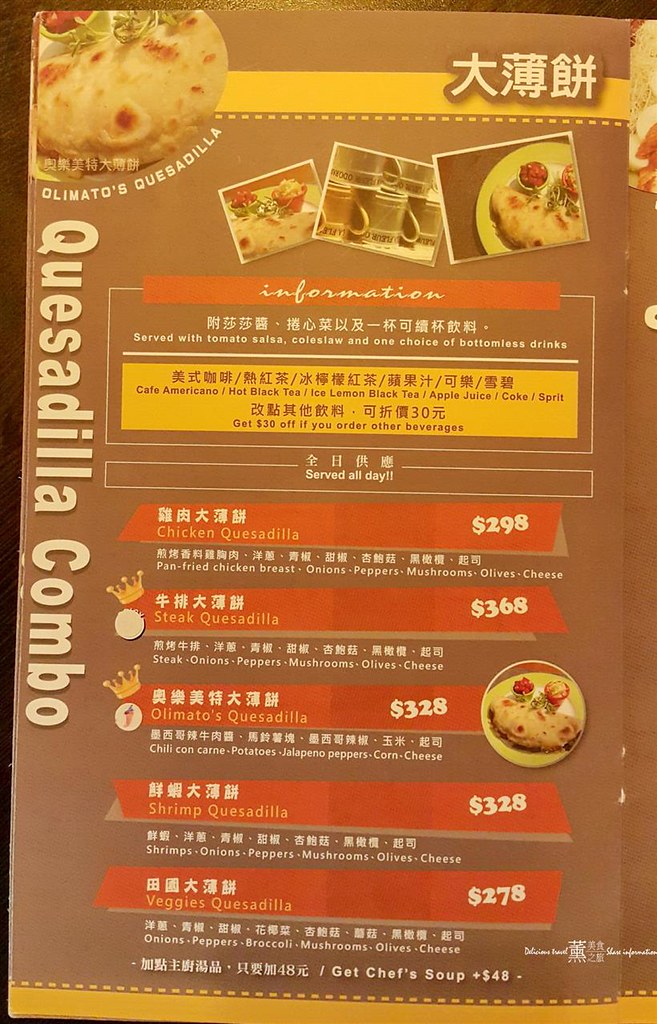This image features a vivid and detailed restaurant menu, presented in both Japanese and English text. In the upper left corner, there is a vibrant picture of a quesadilla, labeled "Olimado's quesadilla." Below this image, three photographs are arranged horizontally: two showcasing mouth-watering quesadillas on the left and right, while the center image displays a neat arrangement of upside-down mugs.

On the left side of the menu, large and prominent text announces the "quesadilla combo." The English text reads as follows:

- "Information" (accompanied by Japanese characters)
- "Served with tomato salsa, coleslaw, and one choice of bottomless drinks"

The available drink options are listed in both languages, including:
- Cafe Americano
- Hot black tea
- Iced lemon black tea
- Apple juice
- Coke
- Sprite

A special offer is noted: "Get $30 off if you order other beverages. Served all day."

The menu details the following quesadilla options:

- Chicken quesadilla: $298 (ingredients: pan-fried chicken breast, onions, peppers, mushrooms, olives, cheese)
- Steak quesadilla
- Olimado's quesadilla
- Shrimp quesadilla
- Veggies quesadilla

Additionally, diners have the option to add the chef's soup for an extra $48. 

The rich imagery combined with the well-organized menu layout invites patrons to indulge in a delightful dining experience.